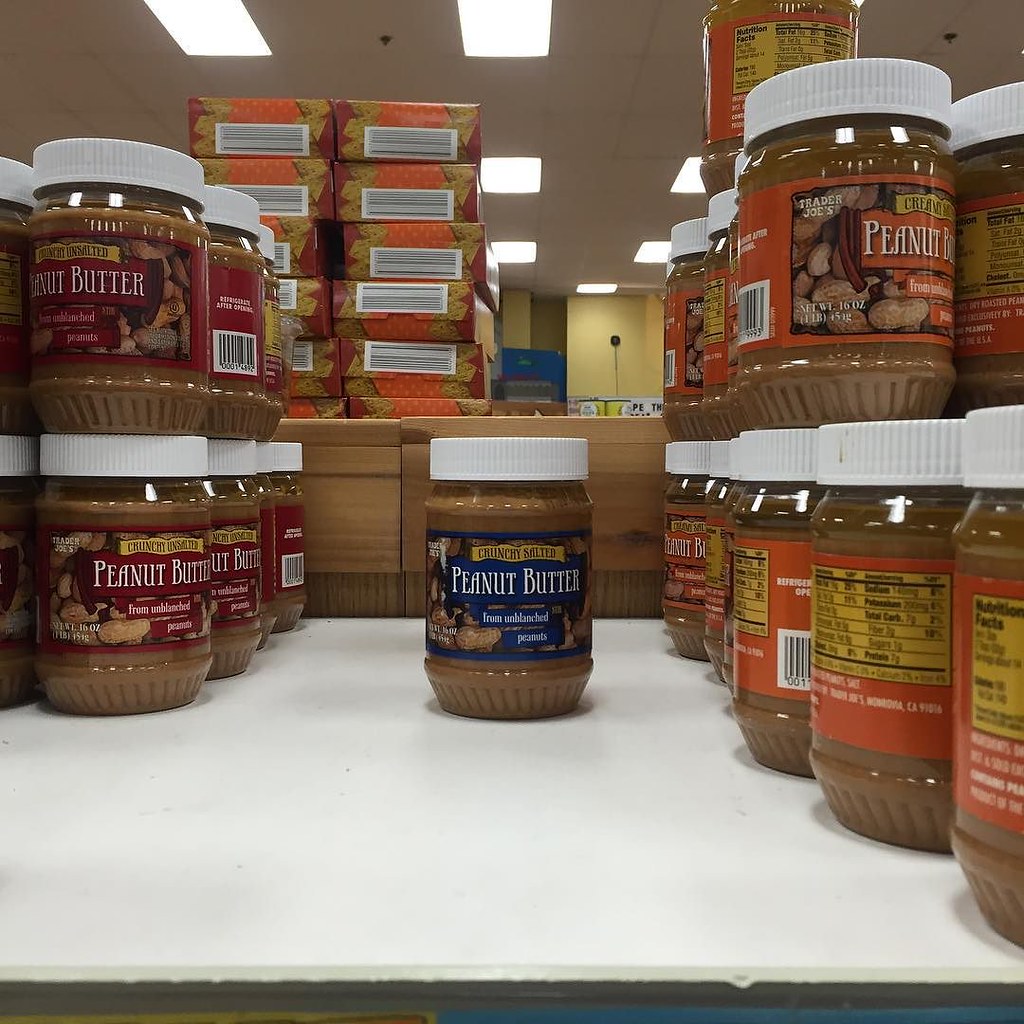This photograph captures a shelf in a Trader Joe's store, lined with an array of peanut butter jars. The shelf itself is white, likely metal, and has some gray smudges and dirt. The jars are stacked two levels high and prominently feature white plastic lids. In the center of the image is a single jar with a blue label proclaiming "Crunchy Salted Peanut Butter from Unblanched Peanuts," accompanied by images of peanuts. To its left, another row of jars features red labels reading "Crunchy Unsalted Peanut Butter," also with peanut graphics. On the right side, jars with orange labels advertise "Creamy Peanut Butter." All jars show the Trader Joe's brand name. In the background, cardboard boxes are partially visible, and the store's white ceiling with fluorescent light panels can be seen at the top of the image.